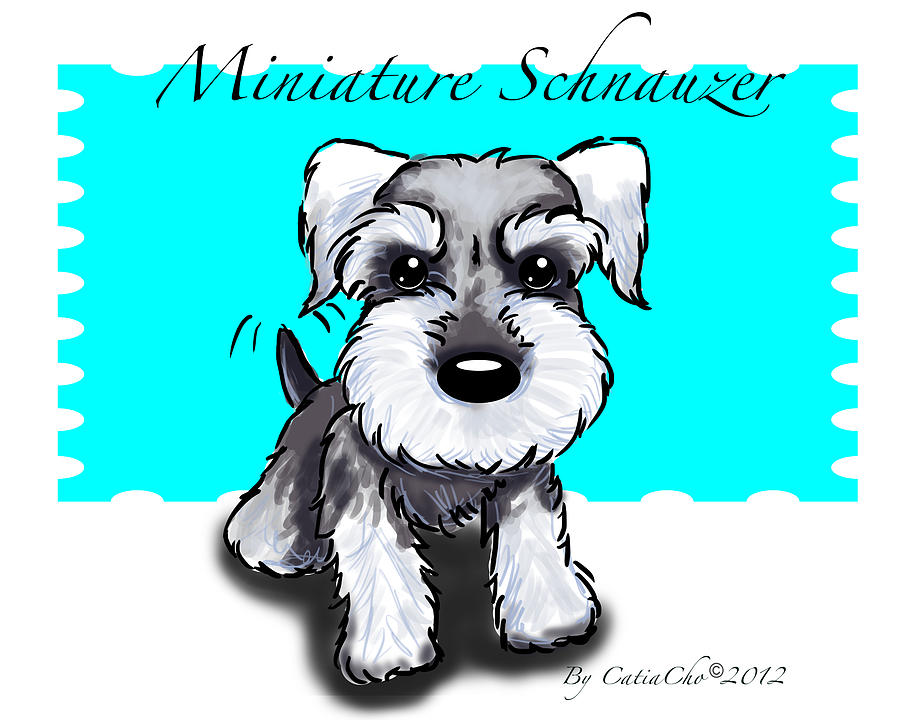The image is a digitally created illustration of a small dog, specifically a miniature schnauzer, rendered in shades of white, black, and gray. The schnauzer is centrally positioned, looking directly at the viewer with its back legs slightly out to the side. It features a black-and-white face with black eyes, white ears, and white eyebrows. Its body and tail are predominantly black, with two black lines on either side of the tail suggesting movement. The background is a light teal (or very light blue) color. At the top of the image, there is black text that reads "MINIATURE SCHNAUZER," and at the bottom right corner, it is signed "by Katya Cho © 2012." The overall image is square-shaped and seems designed for an art website or as a piece of artwork to showcase the artist's skills.